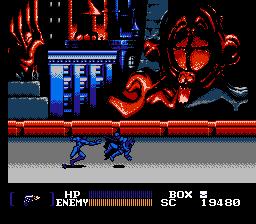This image captures a still from an 8-bit video game, characterized by its blocky graphics and a black frame around the scene. The background features a blue building and a series of indistinct red shapes, including a red wall, set against a gray street gradient that transitions from light gray at the bottom to dark gray at the top. In the foreground, two blue characters are engaged in a combat scenario, with the character on the left appearing to have just thrown a punch, causing the larger character on the right to be airborne, recoiling from the impact. Shadows are depicted beneath each character, enhancing the sense of movement. Along the bottom of the screen, there is a black horizontal bar displaying game statistics in white text: "HP" with a purple health bar and "Enemy" with a yellow health bar. To the right, the text reads "Box" followed by "SC19480".